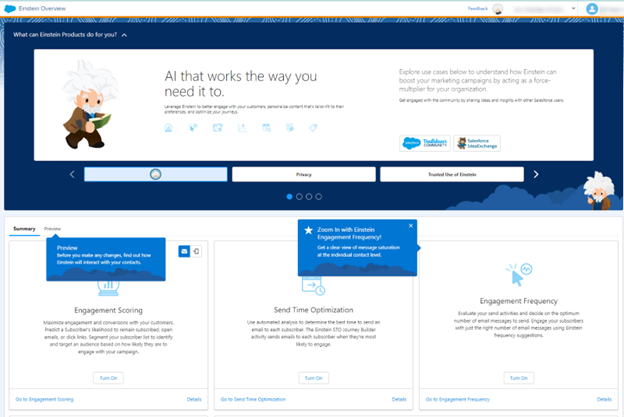This screenshot captures the interface of a laptop application designed for a product that leverages AI to meet specific user needs. The primary background is white, complemented by some blue sections that highlight key features. The application outlines various products and services offered by the company, emphasizing aspects like engagement scoring, send time optimization, and engagement frequency. Additionally, the text invites users to "explore use cases" to learn how this application can enhance marketing campaigns by serving as a force multiplier for organizational efforts. Detailed descriptions and actionable insights are prominently displayed to guide users in optimizing their strategies.